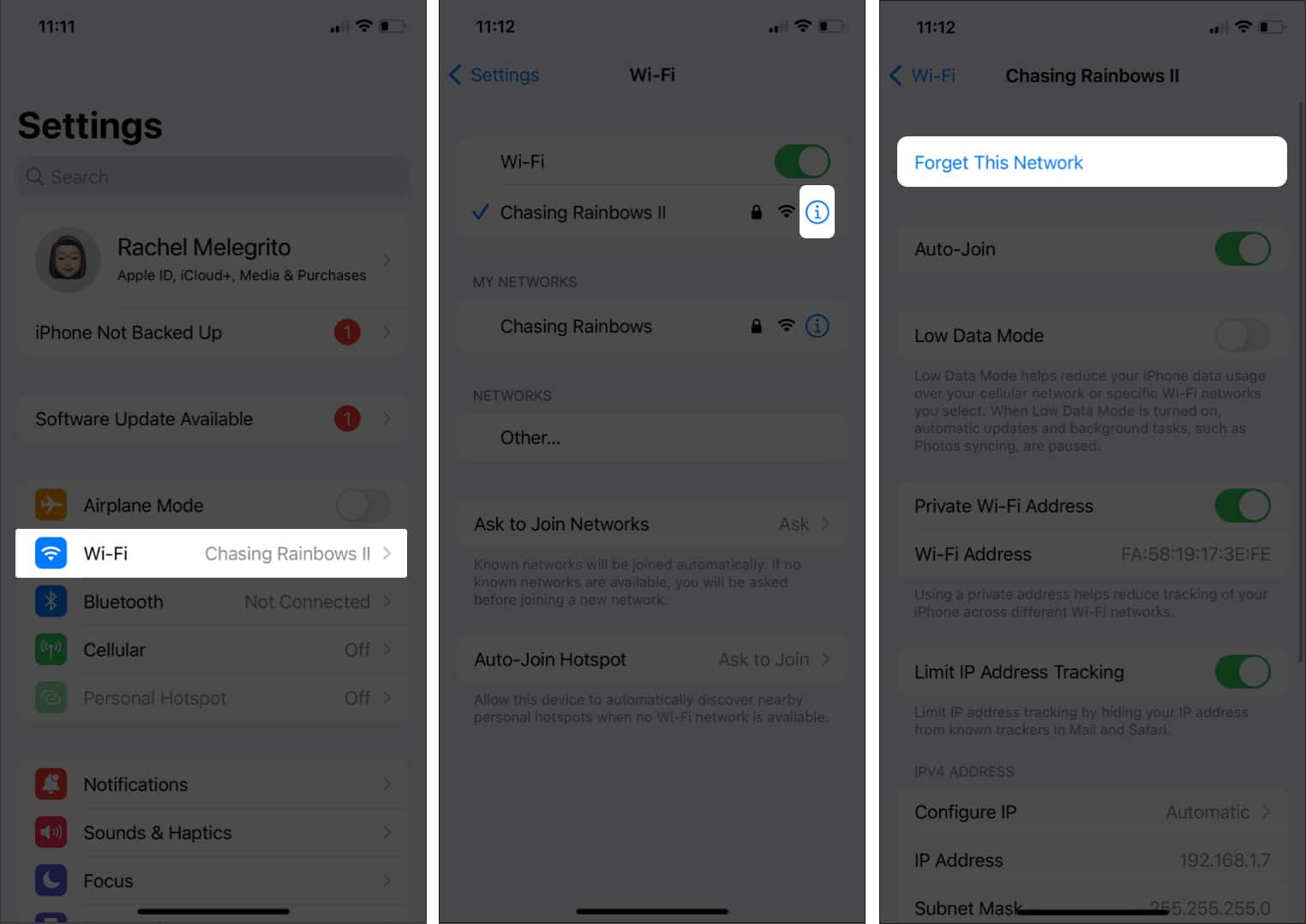The image comprises three side-by-side screenshots displaying various settings on an iPhone. 

1. **Settings Screen:**
   - **Top section:** Displays the current time, battery life, and Wi-Fi status. The heading "Settings" is at the top with a search bar beneath it.
   - **User Information:** Shows the current user, Rachel Melegrito (spelled 'M-E-L-E-G-R-I-T-O'), alongside options for Apple ID, iCloud Plus, media, and purchases.
   - **Alerts:** A red circle with the number 1 next to "iPhone Not Backed Up" and an alert for a "Software Update Available."
   - **Connection Options:**
     - **Airplane Mode:** Slider switched to the left (inactive).
     - **Wi-Fi:** "Chasing Rainbows 2" network is selected.
     - **Bluetooth:** Status is "Not Connected."
     - **Cellular:** Wireless data is turned off.
     - **Personal Hotspot:** Option is grayed out and turned off.
   - **Additional Settings:** Notifications, Sounds & Haptics, and Focus settings are listed with more information options.

2. **Wi-Fi Settings:**
   - **Current Status:** Wi-Fi is enabled with a green indicator and a checkmark beside the selected network "Chasing Rainbows 2."
   - **Details:** Includes a lock icon, Wi-Fi signal indicator, and an informational 'i' in a circle.
   - **Network Options:**
     - **My Networks:** Lists "Chasing Rainbows 2."
     - **Other Networking Options:** "Other," "Ask to Join Networks," and "Auto-Join" options are present.

3. **Chasing Rainbows 2 Network Details:**
   - **Header:** "Chasing Rainbows 2" is prominently displayed with the "Forget This Network" option highlighted.
   - **Settings:** 
     - **Auto-Join:** This feature is enabled.
     - **Low Data Mode:** Not enabled.
     - **Private Wi-Fi Address:** This is selected.
     - **Wi-Fi Address and Limit IP Address:** Specific settings with a slide control available.

This detailed caption outlines each section and feature visible within the screenshots, providing clarity on the settings displayed on the iPhone.